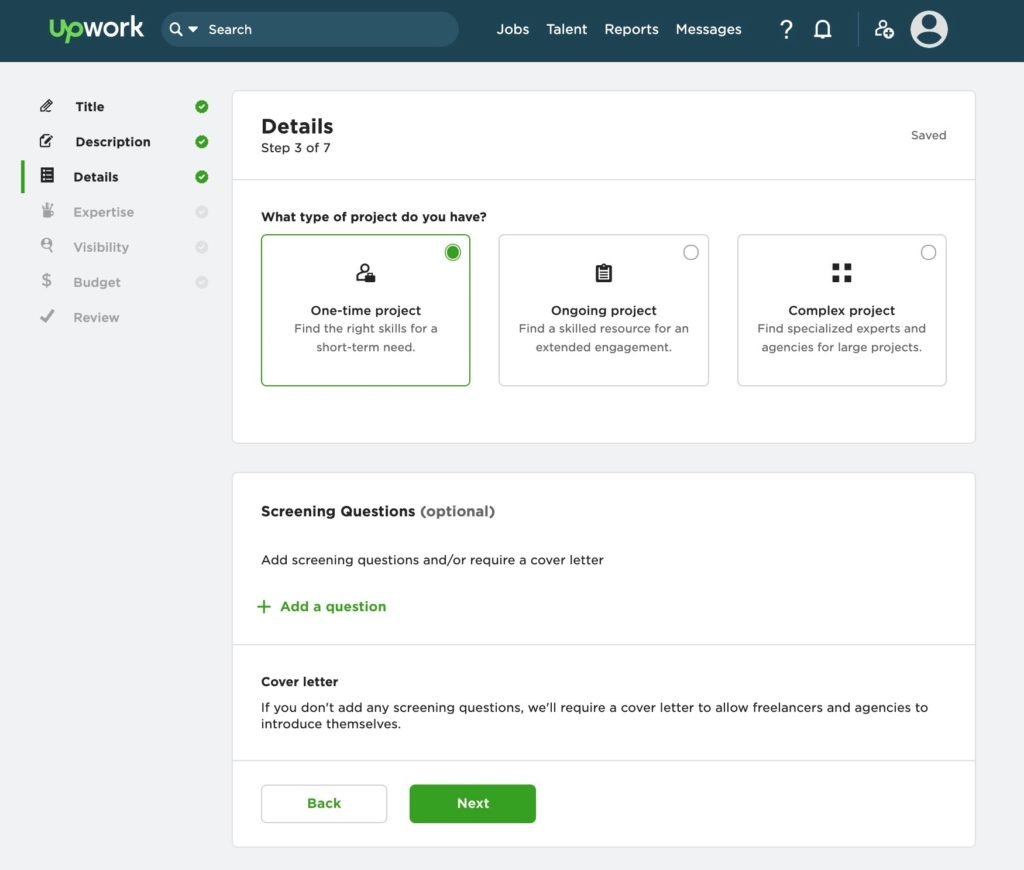This image is a screenshot from the Upwork webpage, characterized by its distinct user interface. At the top, the Upwork logo prominently features the word "up" in green and "work" in white. The header contains a search bar and navigation links labeled "Jobs," "Talent," "Reports," and "Messages," followed by icons for a question mark (help), a notification bell, and user profile options depicted as head-and-shoulders silhouettes within circles.

On the left side of the screen, a vertical menu lists various sections titled "Title," "Description," "Details," "Expertise," "Visibility," "Budget," and "Review." Green check marks indicate completed steps for "Title," "Description," and "Details." 

Center screen, the user is currently on the "Details" section, marked as "Step 3 of 7." Three selectable boxes are displayed under the heading "What type of project do you have?" with "One-time project" selected, indicated by a green circle in the upper right-hand corner of the box. The other options, "Ongoing project" and "Complex project," remain unselected.

Below this, there's a section for "Screening questions" marked as optional, with an option to "Add a question." At the bottom of the screen, the navigation includes a "Back" button and a green "Next" button for progression.

Overall, the image provides a detailed look at the project creation process on Upwork, focusing specifically on the type of project step.